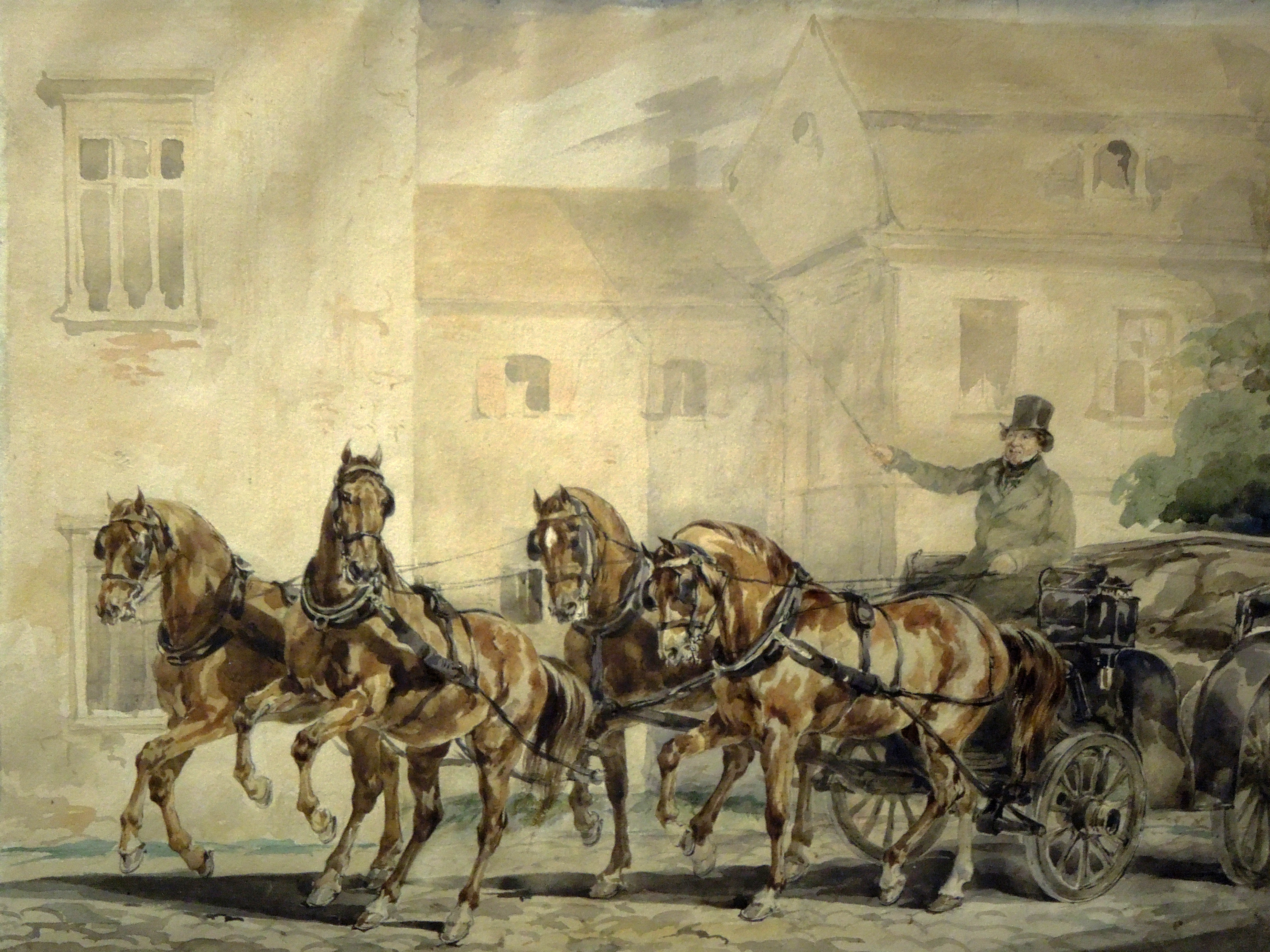The painting depicts an elegant horse-drawn wagon driven by a gentleman, dressed in a top hat and a long buttoned coat. He expertly holds the reins in his left hand and a whip in his right, guiding a team of four beautiful brown horses, each in shades of brown and adorned with elaborate black bridles and collars. The horses appear to be in motion, with at least one of the front horses lifting both front legs as if trotting energetically over a cobblestone street. The wagon itself is refined, with a low back and upholstered seating, highlighted by brown wheels with black centers. The backdrop features a serene, pale beige stone building with a reddish roof, stretching two stories high. The scene is further softened by a foggy, indistinct sky, imparting a tranquil and timeless quality to the artwork.